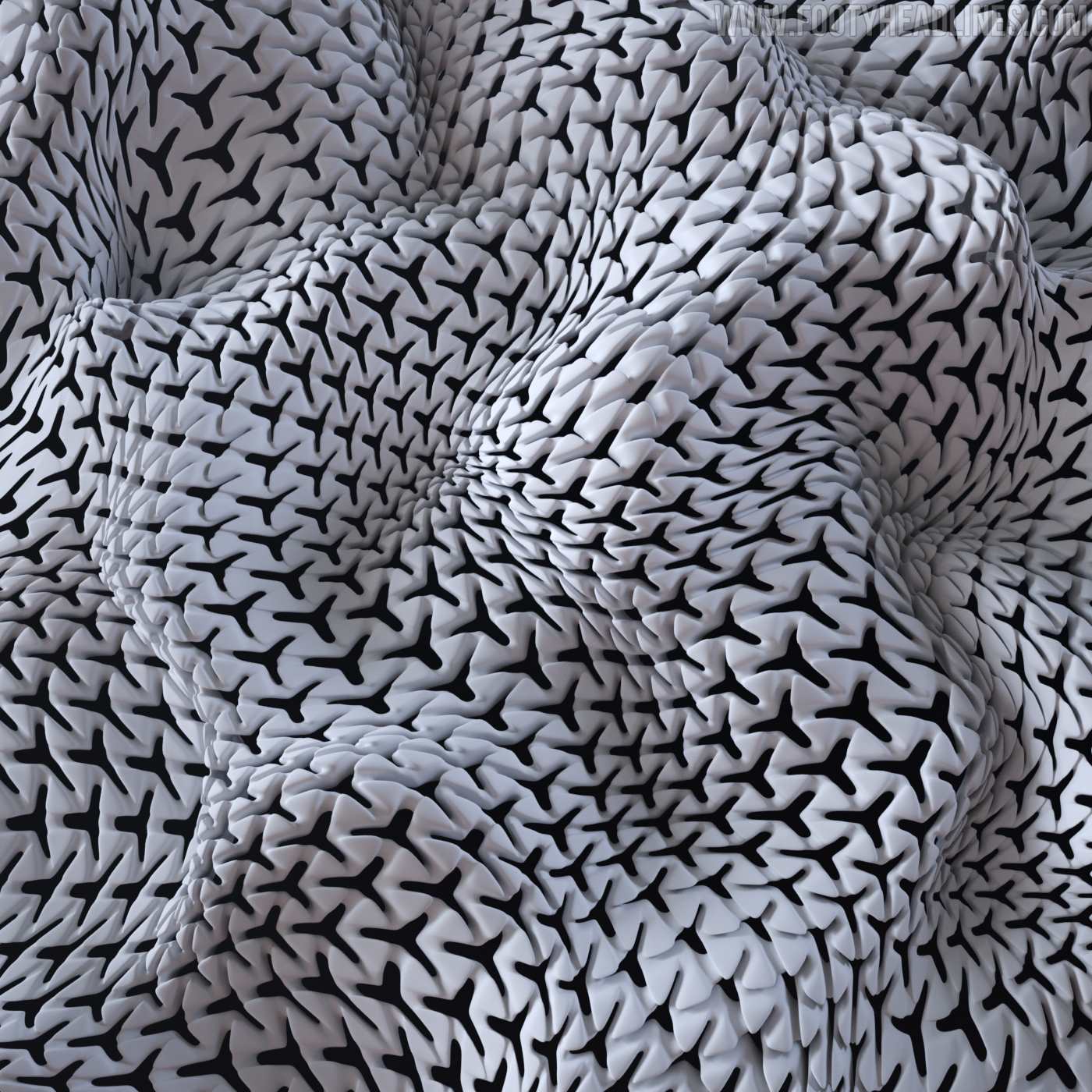A close-up photograph captures the intricate, wrinkled texture of a white fabric, possibly plastic, appearing almost macro or microscope-like. The fabric is crumpled, forming irregular bubble-like shapes that protrude and recede unpredictably. Scattered throughout the image are distorted black shapes resembling three-sided stars or capital letter Y's, evenly spaced yet warped by the underlying folds and ridges. This black-and-white photograph includes shadows adding depth to the texture. A watermark in the upper right corner, barely legible, suggests the image might be sourced from a website, www.footieheadlines.com.